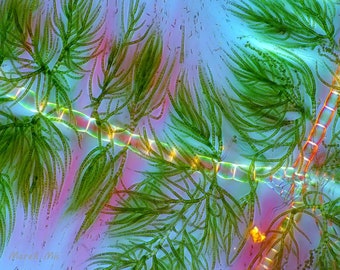The image is a small, horizontal rectangular sketch or painting that combines elements of plant life and underwater scenery, presented almost in a low-resolution, blurry, and microscopic style. Centered in a deep blue and dreamy pink-lavender background are two main chain-like branches, each segment seemingly glowing. One branch extends diagonally from the lower right towards the middle, where another branch diverges and stretches to the far upper left. Both branches are adorned with numerous thin, feathery green leaves that evoke a sense of seaweed or kelp, floating as if underwater or caught in a heavy wind. The green structures display a gradient of dark, medium, and highlighted greens, with small bits of debris or seeds flowing off, adding a dynamic sense to the image. Pink streaks and highlights accentuate the image, especially where the branch segments intersect, imparting an almost ethereal glow. At the bottom right, there's a small, golden heart shape, adding a delicate touch to the intricate composition.